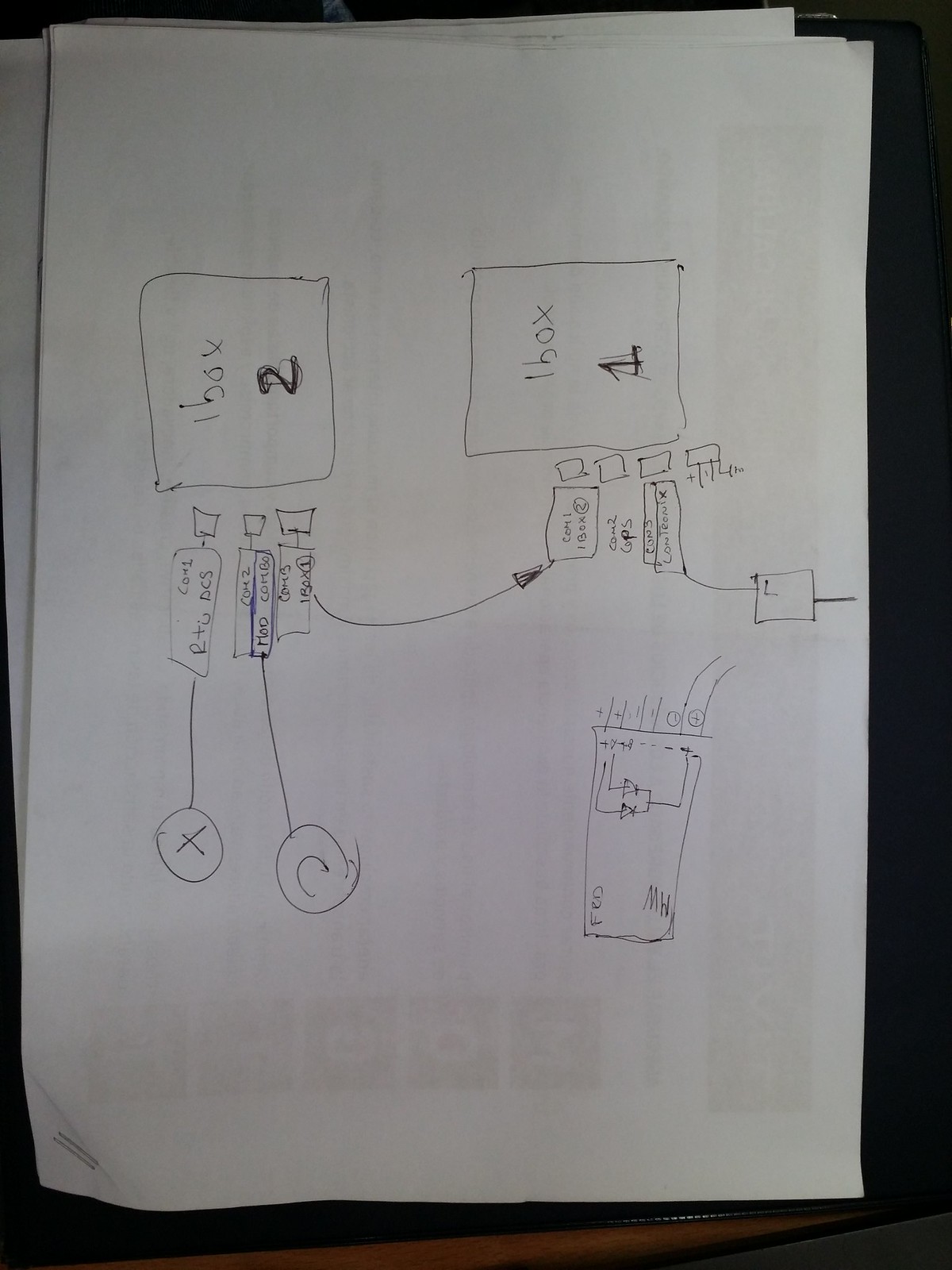This image features a handwritten diagram on a piece of white paper, which appears to be a reused sheet as faint print from the other side is visible. Positioned horizontally, the diagram seems rotated with its left side resting at the bottom, making the right side appear as the top. The diagram is primarily drawn in black ink, with notable inclusion of a blue-outlined square. 

At what is now the top of the image, two square-shaped boxes are labeled "1" and "2", with "2" appearing at the very top. Radiating from the "2" box, are three additional squares. Lines extend from these squares, connecting to a circle with the letter "C" and another circle labeled "X". The intricate arrangement and the utilization of different shapes and colors suggest that this diagram likely represents a complex flowchart or schematic.